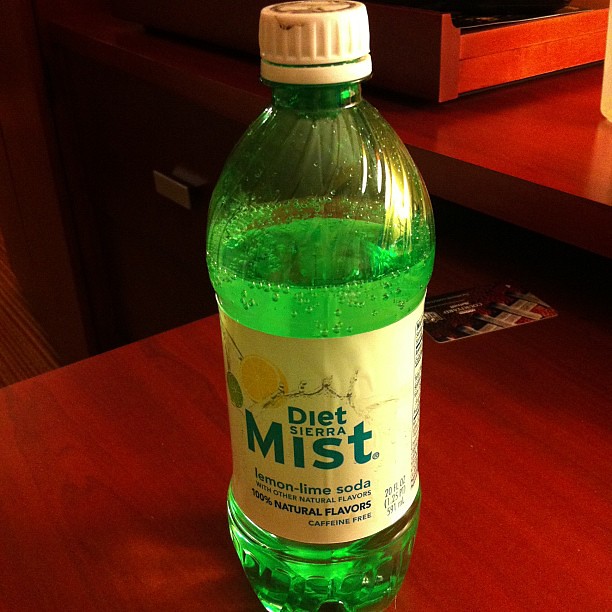A bottle of Diet Sierra Mist is prominently displayed in this image. The bottle is primarily green with a white label, prominently featuring images of an orange and a lime. The label identifies the beverage as a "lemon-lime soda with other natural flavors," boasting "100% natural flavors" and "caffeine-free." The bottle holds 20 fluid ounces (591 milliliters) of soda, which is approximately 75% full, with visible carbonation bubbles. The cap is white, complementing the bottle's color scheme. The bottle is placed on a red, wooden countertop, beside what appears to be a credit card or business card. In the background, there's a glimpse of a wooden object with a metal handle, adding more texture to the setting. The label on the bottle appears to be from an older design, suggesting it is neither very modern nor outdated.